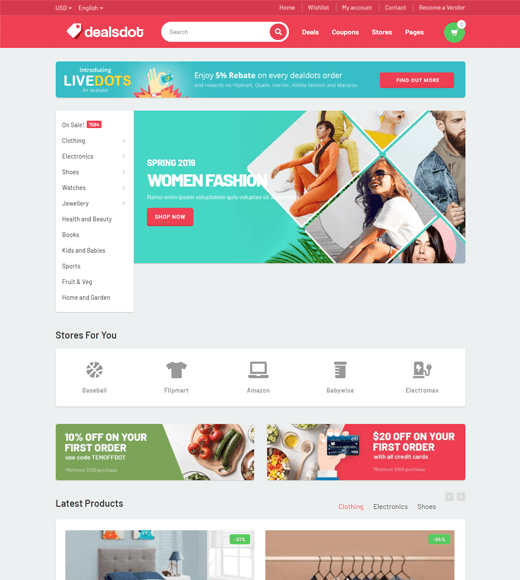Screenshot of the Deals.Dot homepage, featuring a navigation bar at the top. On the left, the website's name "Deals.Dot" is prominently displayed. To the right, a small search bar is positioned for convenient browsing. Adjacent to the search bar, the navigation bar includes section headers labeled "Deals," "Coupons," "Stores," and "Pages." A green circular button with a white shopping cart icon is also visible. Just below the navigation bar, a banner reads "Live Dots: Enjoy 5% rebate on every Deal Dots order." Beneath this banner, there is a promotional section titled "Spring 2019 Women Fashion," showcasing images of three women modeling various outfits, with one appearing to wear a bodysuit.